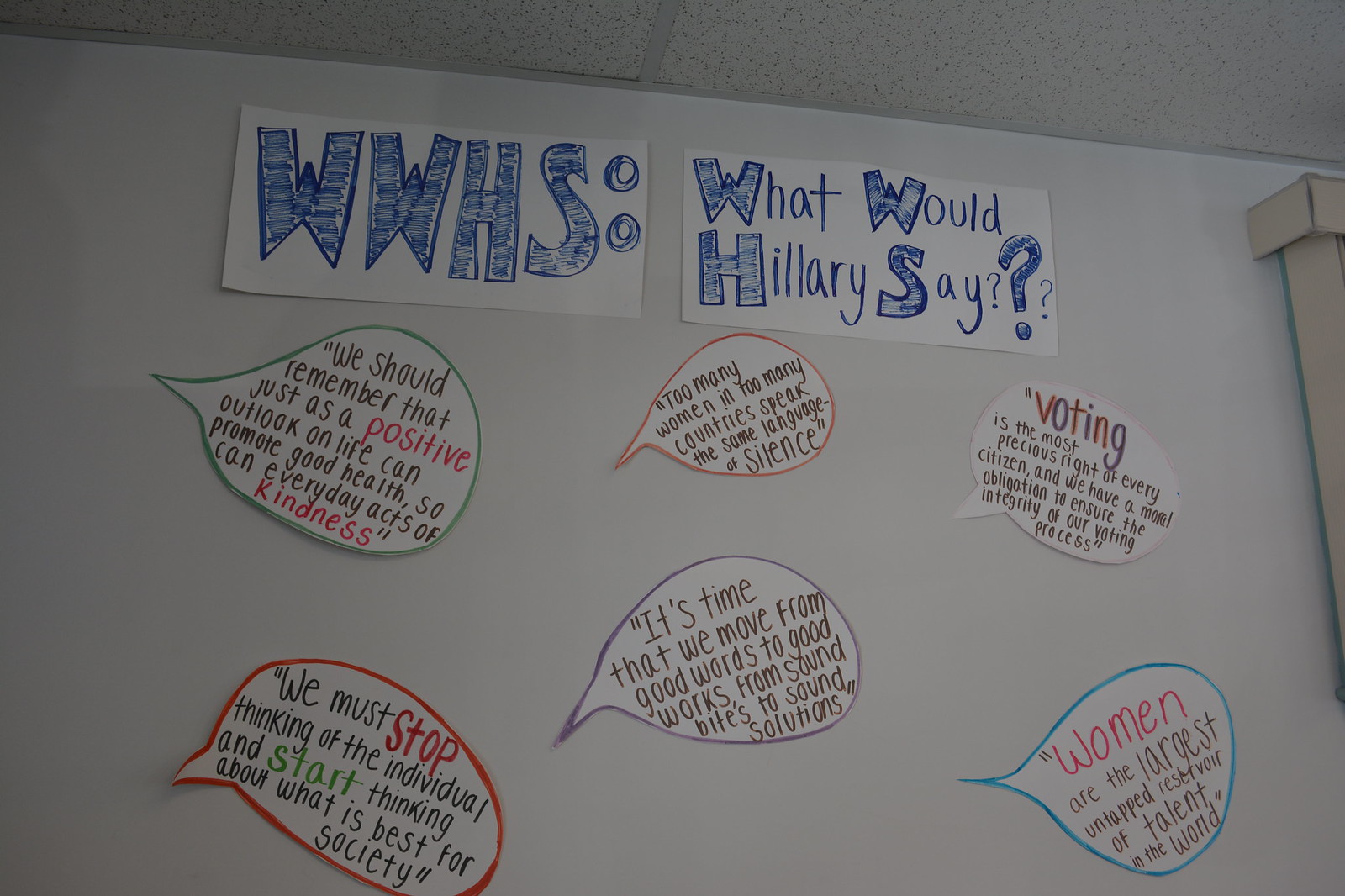The image shows a meticulously designed homemade sign on a white poster board with a thought-provoking message inspired by Hillary Clinton. At the top, "WWHS: What Would Hillary Say?" is prominently written in blue magic marker on white cutout paper. Below this headline are six speech bubbles, each outlined in a different color (green, red, purple, and blue), resembling the kind found in cartoons.

The speech bubbles contain various quotes attributed to Hillary Clinton, each emphasizing important societal and political themes. From left to right, the bubbles convey the following messages:

1. "We must stop thinking of the individual and start thinking about what is best for society," written in black letters with the words "stop" in red and "start" in green, outlined in red.
2. "We should remember that just as a positive outlook on life can promote good health, so can everyday acts of kindness," highlighted by the words "positive" and "kindness" in red, outlined in green.
3. "It's time that we move from good words to good work, from sound bites to sound solutions," framed in a purple outline.
4. "Too many women in too many countries speak the same language of silence," written in black, outlined in orange.
5. "Voting is the most precious right of every citizen and we have a moral obligation to ensure the integrity of our voting process," with "VOTING" displaying alternating blue and red letters, outlined in pink.
6. "Women are the largest untapped reservoir of talent in the world," with the word "women" in red, outlined in blue. 

The white background and wall, along with a partially visible doorframe, emphasize the homemade nature of this bulletin board. The carefully crafted speech bubbles and their meaningful messages reflect a thoughtful homage to Hillary Clinton's ideas and advocacy.